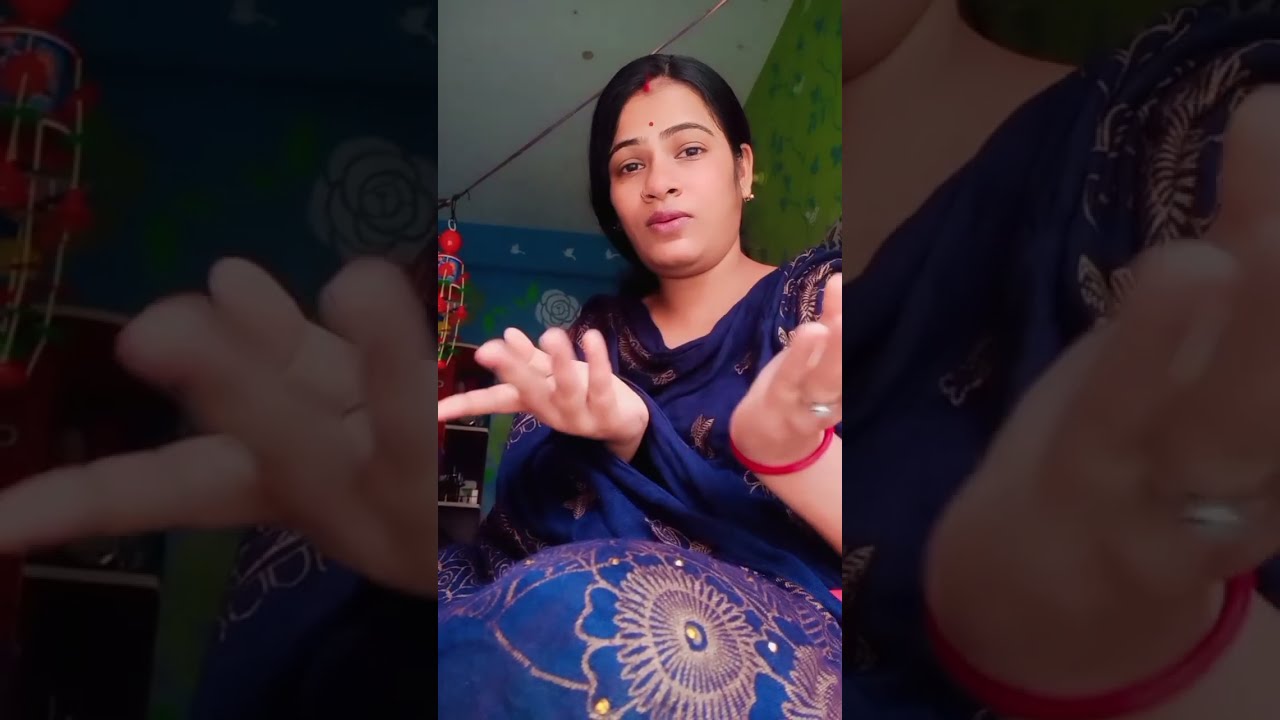In the center of the image is a vertical cell phone photo depicting an Indian woman who has long, dark hair pulled back and a distinct red dot, called a bindi, in the center of her forehead. She gazes directly into the camera with a slightly lowered head, her straight black hair parted on the side. Her dark eyebrows frame her expressive eyes, and her full lips and nose add to her striking features. She's wearing a dark blue dress adorned with a faded gold floral pattern. The dress has no sleeve on the left shoulder. Gold earrings glint in her ears, and a red bracelet adorns her wrist. She holds her hands up, palms facing the ceiling, as if to communicate or present something. 

The background of the image consists of a zoomed-in and faded replica of the same photo, creating a layered effect. This background highlights enlarged sections of her hands and chest area. The setting appears to be a room with multicolored walls; one side is green while the other is blue. A string dangles behind her, featuring a red lantern or decorative object, adding to the rich cultural ambiance of the scene.